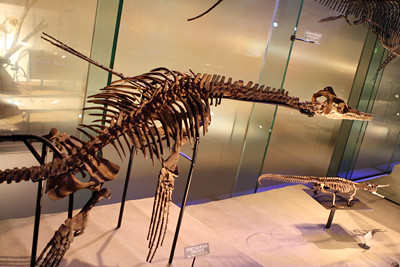The photograph, captured inside a dimly lit dinosaur museum, prominently features a large dinosaur skeleton with a long torso and an elongated neck reminiscent of a smaller giraffe's. The skeleton, including a discernible skull with what appears to be an eye socket, is elevated and supported by metal rods attached to a wooden base. Surrounding the main skeleton are protective glass casings. In the lower right corner of the image, there's a smaller skeleton also mounted on a pedestal. The background reveals glass partitions with translucent qualities, and there seems to be an indistinct object, possibly a tree, visible through the glass on the upper left side. The exhibition setup includes spotlights highlighting the dinosaur skeletons, each labeled with metal name tags identifying the species.